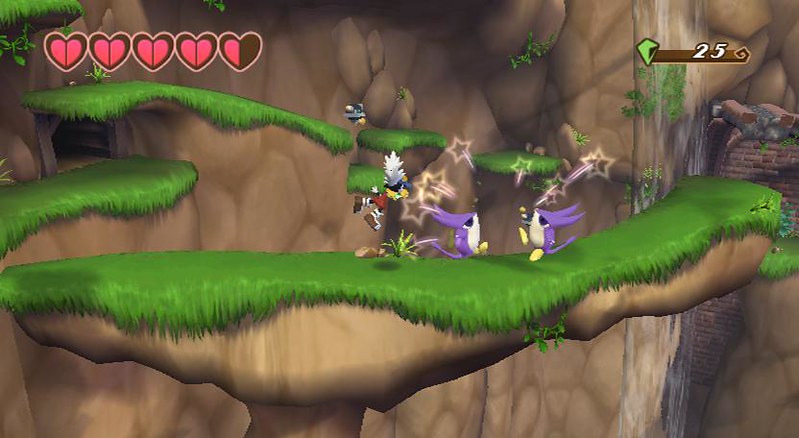The image is a rectangular screenshot from a video game, oriented with the longer side downward. The scene depicts a light brown and whitish background resembling the smoother side of a mountain, interspersed with smaller rock-like edges. Various outcroppings and ledges, fading from light brown to dark brown, are scattered across the mountainside, some covered with flattened grass that overhangs their edges.

At the top of the mountain, two distinct video game characters face each other. Both characters are primarily purple, featuring elongated, horned ears, and white bellies. Their eyes are large and black, and they have yellow feet. Above their heads, faint, white stars can be seen, adding a whimsical touch to the scene.

On the right-hand side of the image, a score indicator displays "25" next to a green diamond, positioned atop a brown surface. Complementing this, the left side of the image showcases five hearts outlined in light pink, presumably representing the player's health or lives.